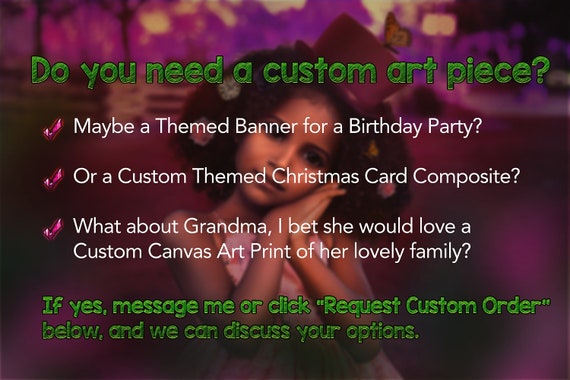The flyer features a young black girl in a predominantly dark purple background. She is striking a charming pose by resting her tilted head against both hands. She is dressed in a pink dress and a purple top hat, though her dark hair is somewhat obscured in the shadows, falling around the nape of her neck. The background hints at vague, blurry images that possibly resemble trees, a bench, or a fence.

At the top of the flyer, bold green text reads: "Do you need a custom art piece?" Below this, a series of three bullet points in white font invite the viewer to consider various custom art options: "Maybe a themed banner for a birthday party, or a custom-themed Christmas card composite. What about Grandma? I bet she would love a custom canvas art print of her lovely family."

The flyer concludes with another green text encouraging engagement: "If yes, message me or click request custom order below, and we can discuss your options."

The vibrant interplay of purple, green, and pink hues in the flyer contrasts against the darker tones, giving the image a uniquely captivating appeal despite the cheesy green font.